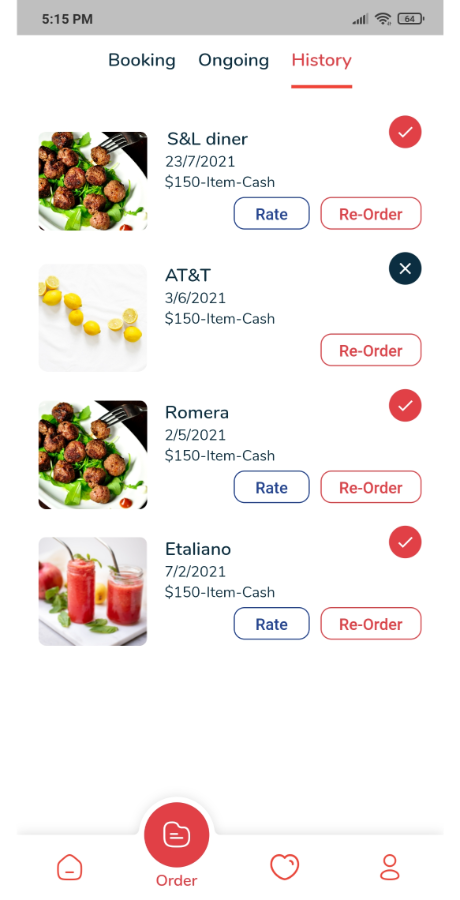This image features a detailed display of various food items available for purchase, organized in a user interface that includes multiple interactive elements. At the bottom of the screen, there's a navigation bar with icons for the order section (currently selected), home, favorites (heart), and user profile, all highlighted in red. 

The top of the screen indicates it is 5:15 PM, with a strong 4-bar cellular signal, perfect internet connectivity, and a 64% battery level. The interface provides options to view ongoing orders or order history, with the user currently in the history section.

The first listing shows "S&L Diner" with an image of meatballs on a plate accompanied by a fork. The item is priced at $23,721 or $150 in cash, and options to rate or reorder are available. An associated red checkmark and a circle with a black X are also visible.

The next entry features "AT&T" offering lemons for purchase at $36,020 or $21 plus $150 in cash, with a reorder option displayed alongside the image of lemons.

Further down, "Romero" appears with an offering priced at $25, $20, or $21 plus $150 in cash. It’s depicted with another image of meatballs on a plate with a fork, and buttons for rating or reordering this item.

Finally, "Italiano" presents an item priced at $7,220, $21, plus $150 in cash, showcased with an image of red smoothies in mason jars. Similar to other listings, users can rate or reorder this item.

Overall, the interface is designed for users to effortlessly navigate, rate, and reorder their past food purchases, with clear visual and textual cues to enhance the user experience.